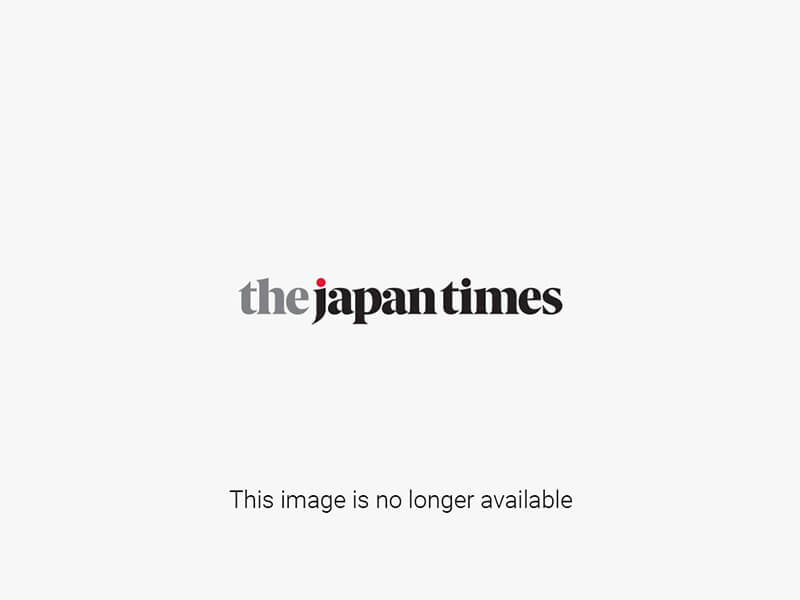The photograph depicts an outdoor scene likely at Tokyo Disney Resort, showcasing a detailed and colorful setting. In the background, the sky is light blue with scattered clouds, casting a serene atmosphere. A prominent brown man-made volcano stands tall, and at its base is a majestic white castle adorned with various gold domes and towers. 

The foreground captures a unique moment: a woman in a blue silk kimono with white and yellow floral patterns, and a red and white flower decoration in her hair, is taking a photograph of a small group of people. These individuals, all sporting face masks and appearing to be of Asian descent, are posing for the camera with smiles hidden but visible through their eyes. The group consists of three girls standing in elegant kimonos complemented by white fur stoles, and two boys kneeling in sharp suits, each holding a plastic bag with the Mickey Mouse logo and “Tokyo Disney Resort” inscription. Surrounding them is a large courtyard paved with textured gray stone blocks, bustling with other visitors.

This vibrant image is bright, clear, and well-lit by natural sunlight, capturing not just a photograph but the joy and essence of an idyllic day spent at a captivating location.